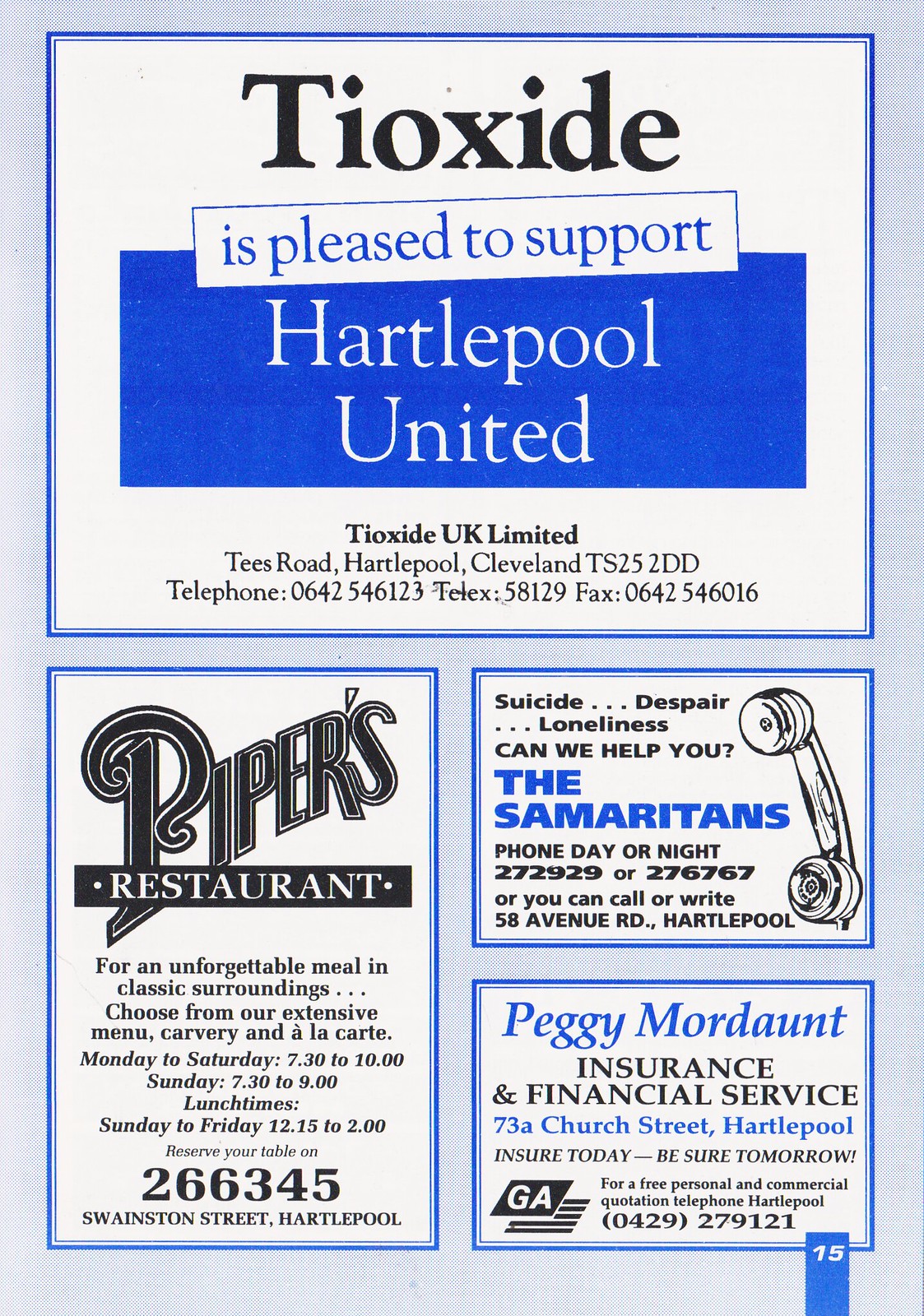The image is a page seemingly from a magazine, primarily featuring advertising content. The main ad at the top, bordered in blue, displays a large white box with bold black text stating "Tioxide is pleased to support Hartlepool United," with "Hartlepool United" prominently displayed in white text against a blue background. Below this, in smaller black font, the contact details for Tioxide UK Limited are provided, including their address in Hartlepool, phone number, telex, and fax number.

Beneath this primary advertisement, there are three smaller horizontal rectangles stacked vertically and horizontally. The ad on the left features "Piper's Restaurant" written prominently in black text on a white background. It describes the restaurant's offerings, including an extensive menu with Carvery and a la carte options, and lists operating hours: Monday to Saturday from 7:30 to 10, Sunday from 7:30 to 9, and lunchtimes Sunday to Friday from 12:15 to 2. The ad concludes with a reservation contact number and the restaurant's location on Swanson Street, Hartlepool.

To the right, the top rectangle addresses issues of "suicide, despair, loneliness," asking if help is needed, with "The Samaritans" printed in blue ink next to an image of a phone receiver. Below, it provides their contact details for day or night assistance, including a phone number and their address on 58 Avenue Road, Hartlepool.

The bottom-right rectangle features "Peggy Mordant" in blue ink, followed by "insurance and financial service" in black. Below, an address in blue ink specifies 73A Church Street, Hartlepool. The ad concludes with a tagline "insure today, be sure tomorrow" and provides a contact number for quotes and services.